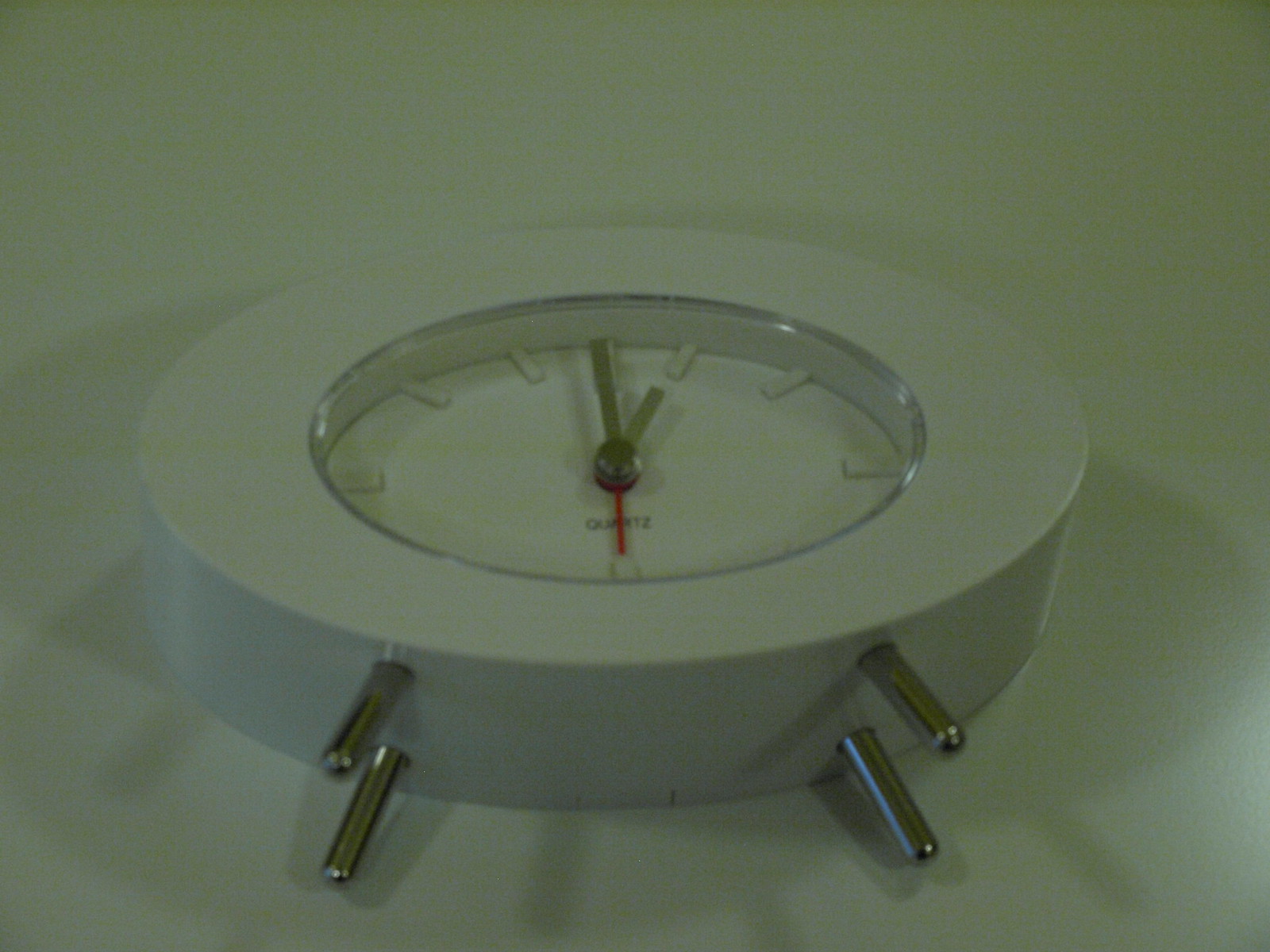This image depicts a round, analog clock lying on its back. The clock has a diameter of approximately 8 to 10 inches and features a thick white or cream-colored plastic edge. A silver inner ring frames the face of the clock, which matches the hue of the edge in its white or cream shade. The clock's face is adorned with green hour and minute hands, while the second hand is strikingly red. Notably, the clock is positioned on its back, supported by four silver metal legs that would typically stand it upright. This detailed arrangement highlights the design and color contrast of the clock components.